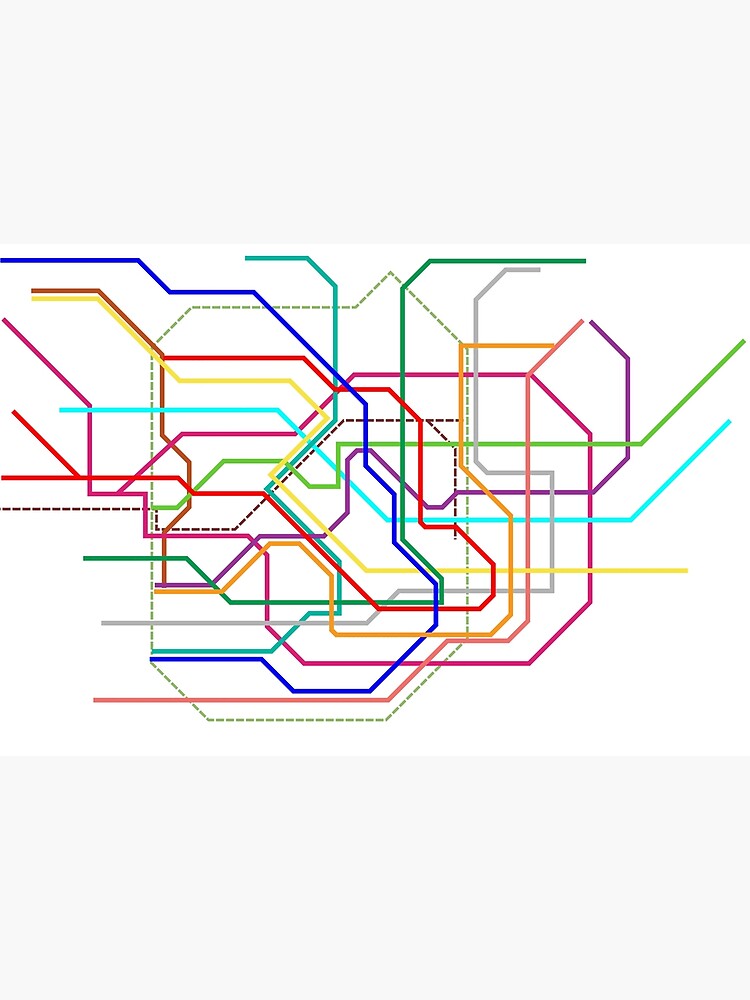This image is a detailed, colorful diagram, potentially illustrating a transportation system, circuitry wiring, or telephone wiring assembly. The diagram is set against a white background with a gray border at the top, transitioning to white about one-third of the way down. Various solid and dotted lines, each uniquely colored, crisscross and intersect at different angles throughout the image. The colors include vibrant shades of green, teal, blue, purple, orange, red, yellow, royal blue, pink, magenta, and brown. Some lines are dotted in deep brown and lime green. The lines intertwine intricately, suggesting complex pathways or connections, emphasizing an organized yet intricate network. The overall composition lacks any textual information, leaving the exact identification of the diagram open to interpretation.